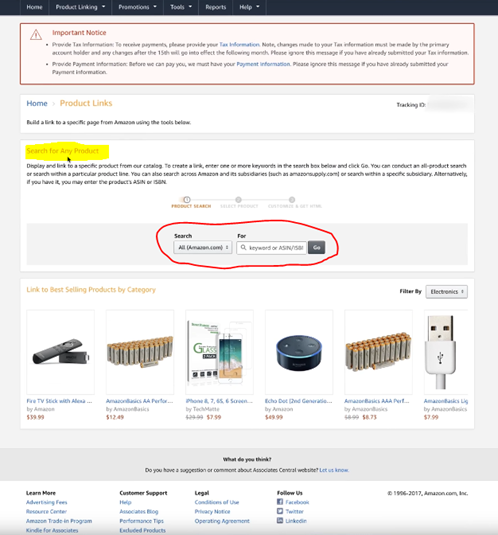This image is a detailed screenshot of an Amazon seller dashboard page. At the top of the page, a black navigation bar displays various menu options such as Home, Product Listing, Promotions, Tools, Reports, and Help. Directly beneath this bar is a prominent red box labeled "Important Notice," which includes a red triangle with an exclamation point inside, signaling a significant alert.

Immediately below, there is a section titled "Home" followed by "Product Links." This area is highlighted in yellow and includes the text "Search for Any Product." Further down the page, the dashboard displays six products. At the top left of this product section is the text "Link to Selling Products by Category,” and on the right side, there is an option to filter products by Electronics. 

At the bottom of the page, four columns of blue links offer additional navigation options. The layout and color coding (including the significant use of red and yellow) enhance usability and draw the user's attention to key areas of the dashboard.